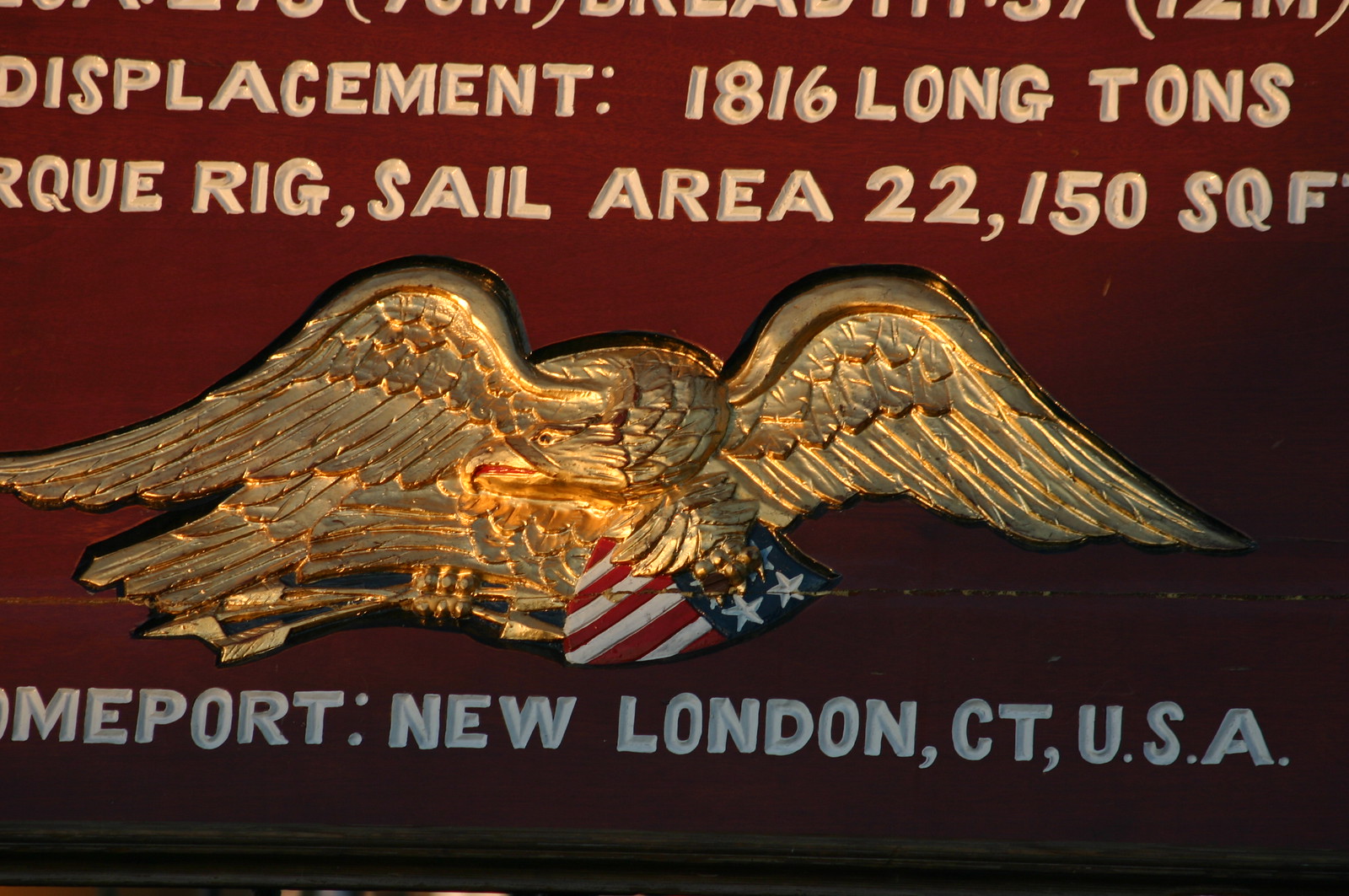The image features a zoomed-in view of an elaborately designed emblem. Dominating the center is a gold American eagle, carrying two arrows and a shield, all set against a rich burgundy red background. Above the eagle, in white letters, are the words "displacement 1,816 long tons." Part of a word, ending in "QUE," is also visible, followed by the phrase "rig, sail area 22,150 square feet." Below the eagle, there's the text "HOMEPORT: New London CT USA." The sign is bordered by a black frame. The gold text, slightly less vibrant than the eagle but still within the same color family, provides statistical details that are partially obscured due to the zoomed-in nature of the image.